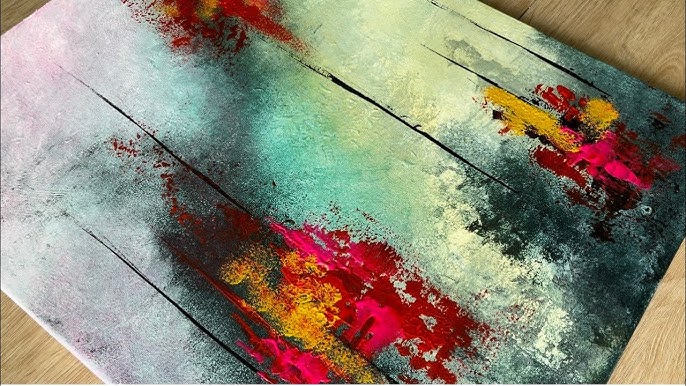The photograph depicts a small, colorful rug placed on a hardwood floor. The image is taken from above, closely cropped so that the edges of the rug extend out of the frame, revealing only parts of the wooden floor around it. The rug features an abstract design with an array of vibrant, shiny, metallic-like colors. In the upper left, lighter purple hues transition into darker shades, complemented by streaks of red and orange in varying intensities. The middle section showcases a blend of yellow, orange, and red while the lower right corner shifts from lighter to darker blues with hints of green. The colors, including red and yellow, also appear in the upper right-hand corner though just barely within view. The rug's surface has a bright, glossy appearance, creating a visually striking and shiny effect akin to metallic finishes.